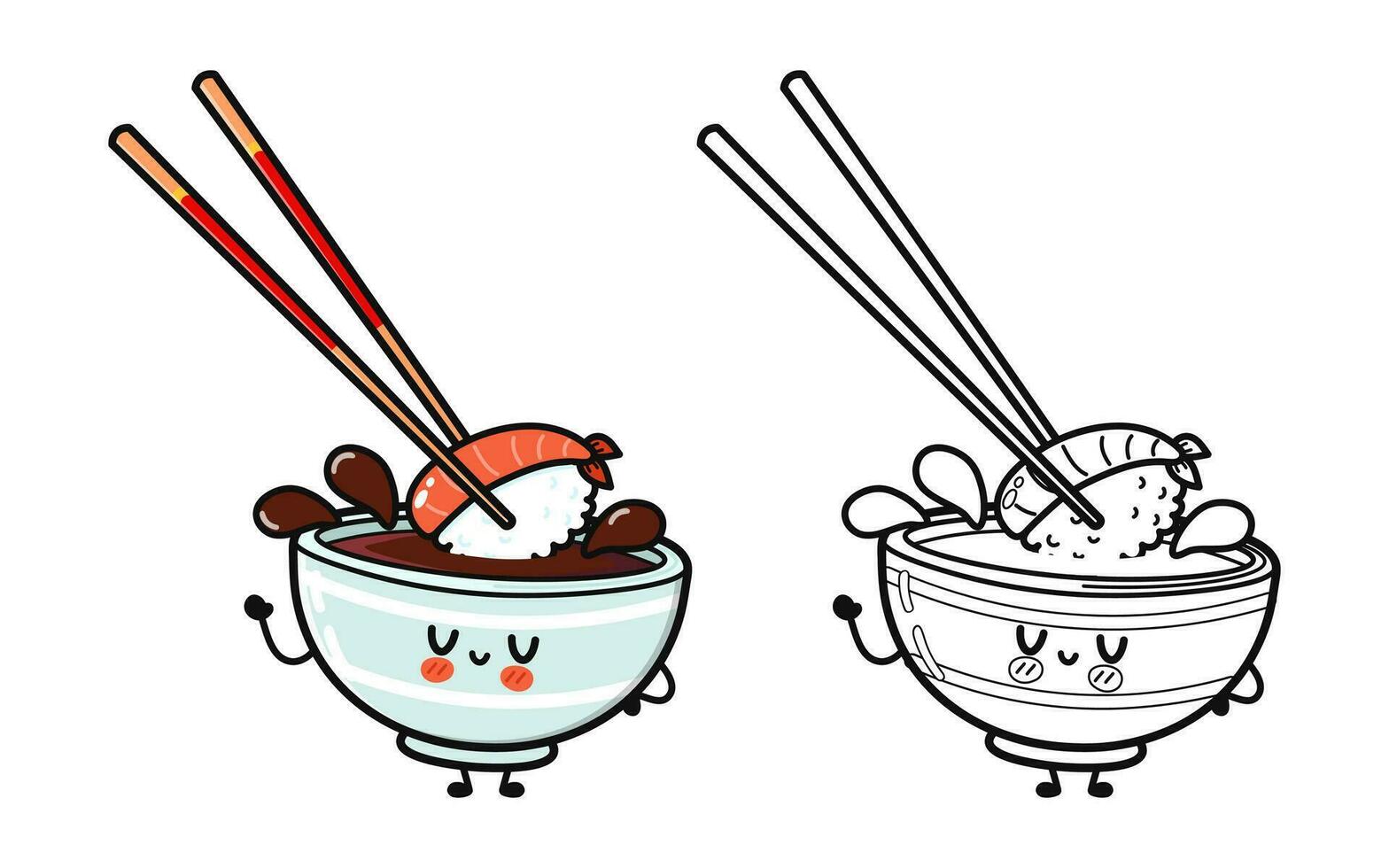This whimsical digital artwork presents two versions of the same delightful scene: one in vibrant color on the left and a black-and-white sketch on the right. The centerpiece is a cute, personified cup with a light blue hue featuring adorable facial features, including closed eyes, a cheerful smile, and rosy cheeks. The cup also sports stubby little legs and delicate arms. Two wooden chopsticks with hints of red and yellow delicately grasp an orange piece of sushi, dunking it into the cup's contents, which resemble hot chocolate or coffee. The colored version reveals the nuanced details, with horizontal lines adorning the cup, while the sushi and chopsticks are distinctly orange and tan respectively.